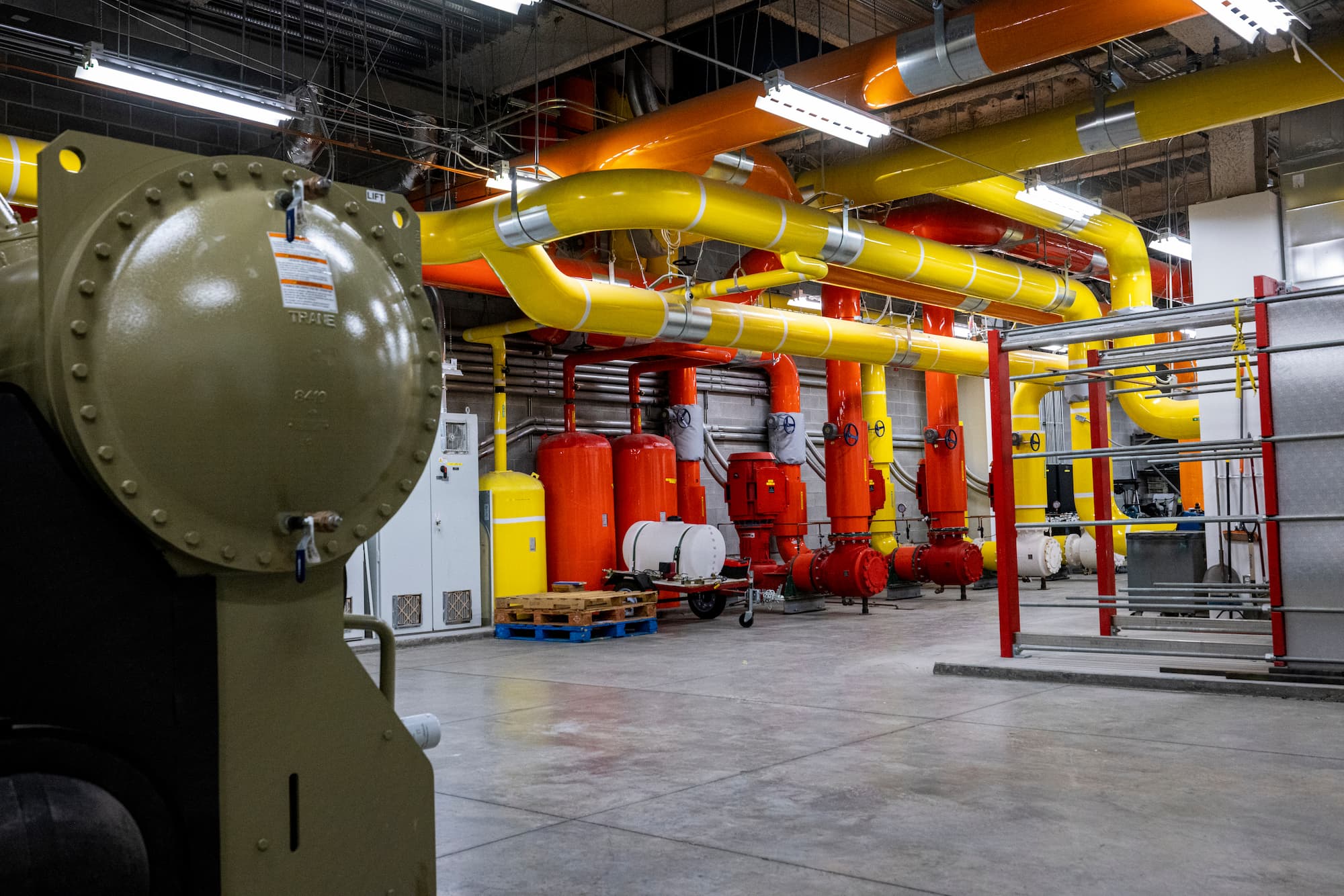The photograph depicts the interior of an industrial building, resembling a basement due to its exposed rafters, unfinished ceiling, and visible pipes. The dominant feature is the intricate network of colorful piping—primarily yellow, orange, and red—that winds its way across the ceiling and into the depths of the space. Prominent in the central and upper portions of the image, these pipes connect to large cylindrical boilers in similar colors. There are three notable boilers: two red ones and a smaller yellow one, positioned towards the center left. These vivid hues contrast against the gray concrete floor and the surrounding gray walls. In the foreground, to the left, sits an olive-green, circular mechanism atop a console, partially cropped by the photograph’s frame. This device is adorned with rivets and adds to the industrial essence of the scene. Additionally, a box housing fans, possibly a circuit box, is visible beneath the boilers. Scattered pallets and steel rods hanging from a red base further enhance the industrial ambiance of the image. Ceiling lights cast a muted illumination over this meticulously detailed industrial environment.